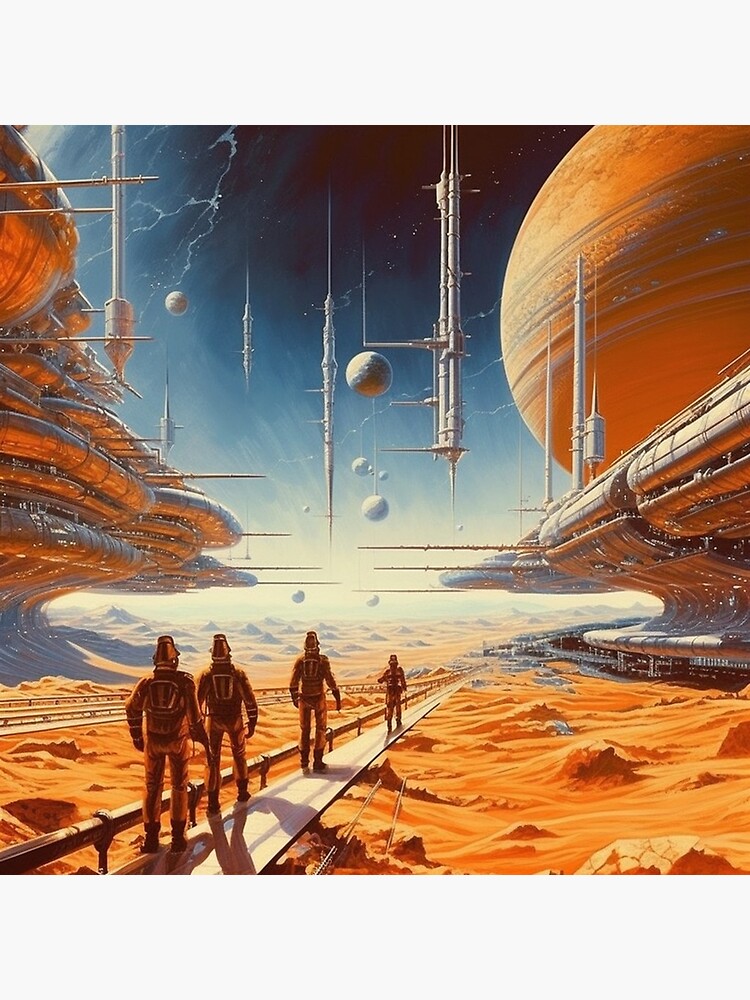The artwork, seemingly generated by AI, presents a detailed and vivid futuristic space scene, featuring a barren, rocky landscape reminiscent of Mars. Dominating the upper right portion of the image is a large orange planet, beneath which a silver spacecraft is positioned. Surrounding the orange planet are multiple silver globes and elongated silver cylinders, adding to the otherworldly atmosphere. On the left side of the painting, another orange-colored spacecraft can be seen, contributing to the futuristic theme. The bottom of the painting showcases an orange-hued landmass, with jets of some sort positioned upwards at intervals. Cutting through the landscape is a long, winding road or pavement. Along this path, four figures in coppery-orange uniforms march forward. The uniforms are complete with gloves, metal bucket-like helmets, and backpacks, emphasizing their roles as spacemen or explorers in this advanced setting. Off in the distance, needle-like structures and shiny spheres hint at the presence of additional futuristic buildings or habitats, suggesting a detailed and inhabited extraterrestrial environment.